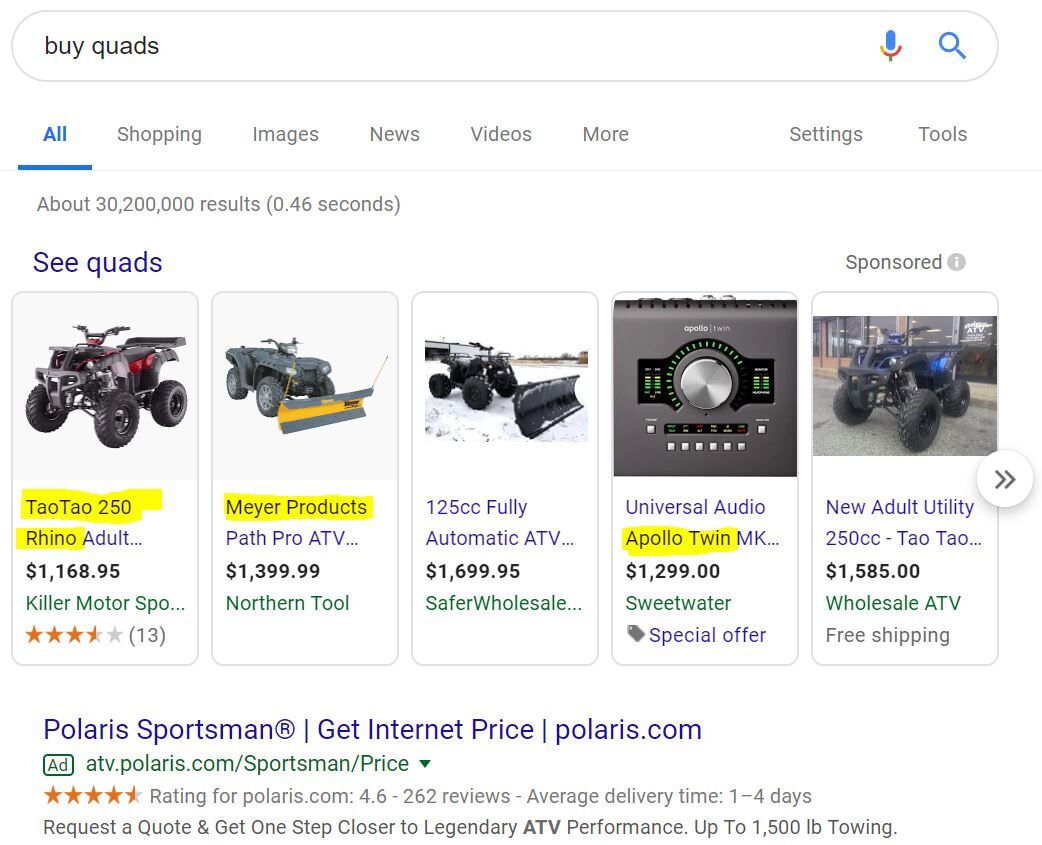The image depicts a search engine page where the query "buy quads" has been entered into the search box at the top. Just below the search bar, navigation options are visible, such as "All," "Shopping," "Images," "News," "Videos," "More," "Settings," and "Tools." The search results indicate there are approximately 30,200,000 results, fetched in about 0.46 seconds. The initial section showcases sponsored posts featuring different quads.

The first result shows a black and gray quad with red accents, labeled as "TauTau 250 Rhino Adult" priced at $1,168.95, offered by Killer Motorsports, and has a rating of 3.5 stars from 13 reviews.

The second featured quad is equipped with a snow plow at the front, identified as "Meijer Product Path Pro ATV" with a price tag of $1,399.99 from Northern Tool.

The third listing also displays a quad with a plow, showcased in a snowy environment. This model is a "125cc fully automatic ATV" priced at $1,699.95 from Safer Wholesale.

At the bottom of the search results, there's a link to the Polaris Sportsman series, with a prompt to "get internet price" on Polaris.com.